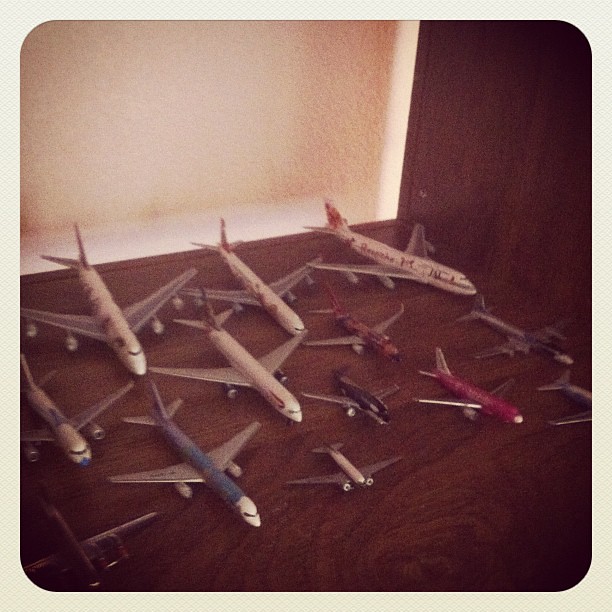This detailed photograph captures an intricate display of model airplanes arranged on a brown wooden floor with a rich, red hue, set against a stark white wall. The collection is meticulously organized in rows descending in size. In the back, closest to the wall, are three large model passenger jets, primarily silver and white, with some displaying varied colors, including blue and red. In front of these are smaller commercial aircraft, with a tiny black one among them. The front rows showcase even smaller models, including military aircraft that appear to date back to the 1950s, with some featuring propellers and others jets. The variety significantly reflects both commercial airliners like the 747 and military planes, with a biplane among the mix. Additionally, a wooden door can be seen to the right, grounding the scene in a cozy, lived-in space.